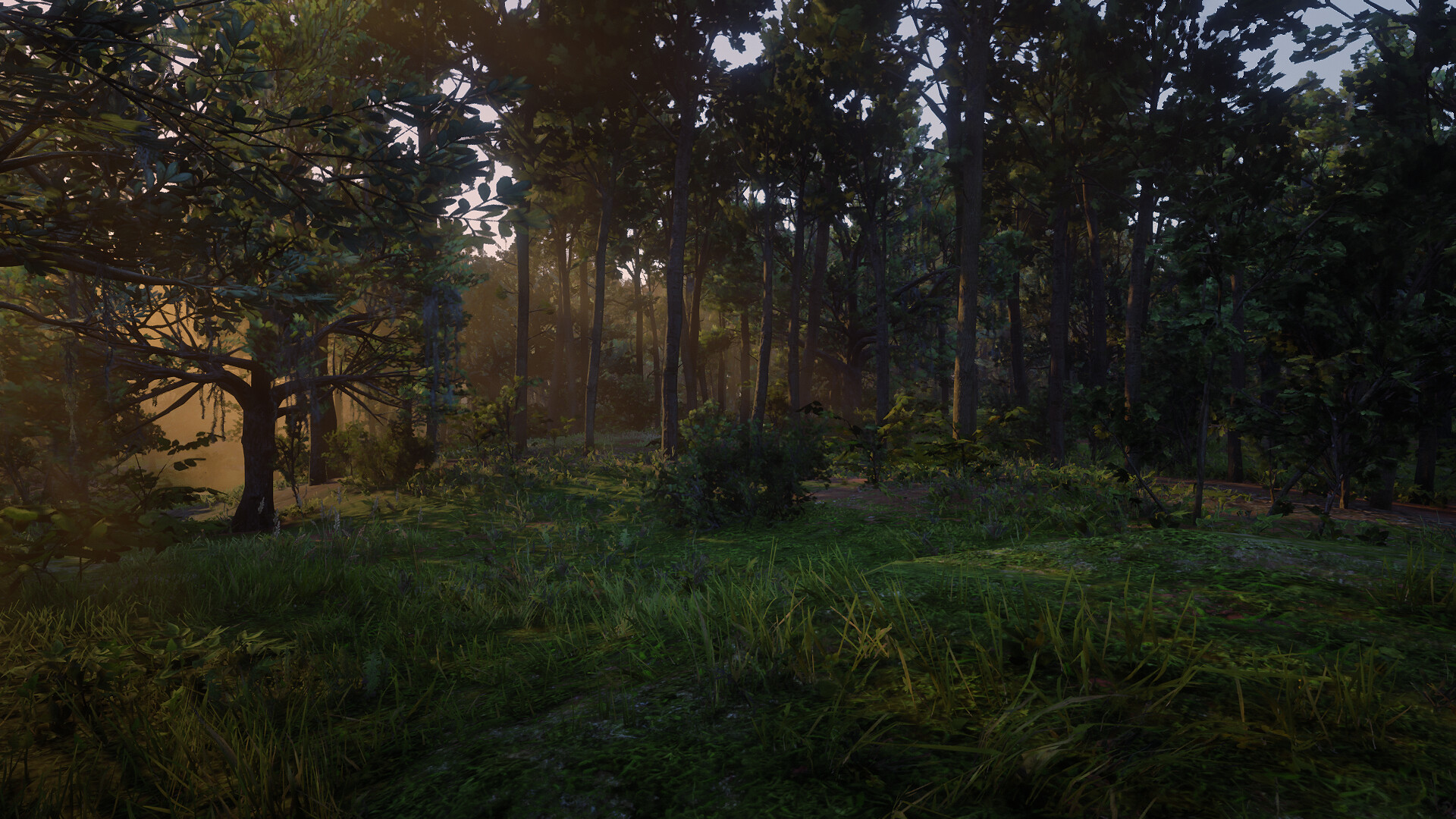A panoramic view of a dense forest captures the serene beauty of nature with lush greenery and a variety of plant life. The ground is covered with green grass, varying in height from patches of tall blades to shorter, more even sections. Interspersed among the grass are different types of plants, predominantly green, though some areas reveal brown earth and sparse vegetation. The forest is filled with a multitude of tall, slender trees, their trunks a healthy brown. The trees are adorned with abundant foliage that transitions from vibrant yellow to rich green, and into deeper, darker hues depending on the lighting. From the left edge of the image, the sun peeks through, casting its early morning or late afternoon glow over the forest, suggesting the sun is either rising or setting just beyond the horizon, illuminating the scene with a warm, gentle light.